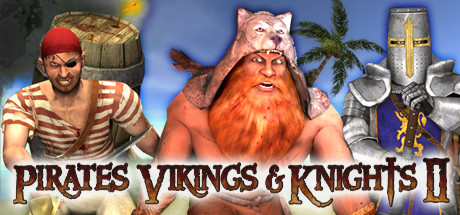This image is a digitally animated horizontal rectangle, likely an advertisement or banner for a video game or cartoon titled "Pirates, Vikings, and Knights II" displayed in brown text with a white glow at the bottom. The scene is set outdoors with a blue sky backdrop and a palm tree. The composition features three distinct, waist-up male characters spanning the width of the image. On the left stands a pirate with a white complexion, grimacing expression, wearing a red bandana and black eyepatch, a red and white striped shirt, white pants, and carrying a wooden barrel on his back. In the center is a shirtless Viking, characterized by his full red beard, lightened skin, and a helmet fashioned from a wolf's head. He is depicted in brown pants. On the right, a medieval knight is clad in stainless steel armor with a blue chest cloth, black gloves, and a helmet featuring a gold cross on the front. He holds a shield adorned with a purple and gold emblem. The detailed digital artwork collectively highlights each character's distinctive historical attire and persona, set against the vibrant outdoor backdrop.